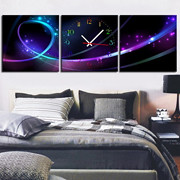The image depicts a small, color photograph of a modern bedroom featuring a double bed with a bedspread draping down the right-hand side and a cushion placed at the bottom left corner towards the foot of the bed. The bed is dressed in a combination of dark gray and white linens, including a dark gray comforter, a light gray accent pillow, dark gray pillowcases, and a black and white plaid blanket. Above the bed, there is a piece of three-part artwork split vertically into equal sections, presenting a continuous, vibrant, and futuristic outer space theme with swirls of pink, purple, turquoise, and hints of yellow. The central piece features a clock face, with the little hand just above the ten and the right hand just above the two, indicating the time is approximately eight minutes past ten. A nightstand beside the bed hosts a lamp and possibly a cup, adding to the room's cozy yet contemporary ambiance.